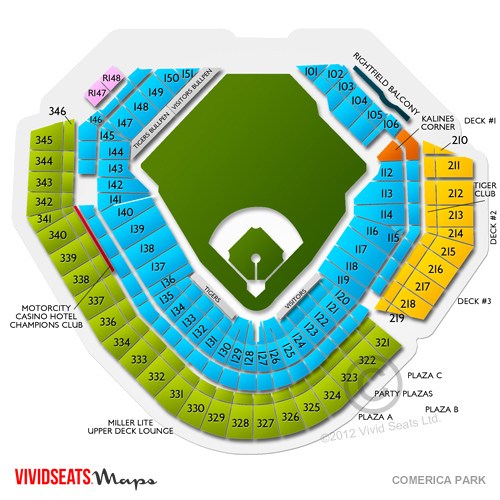This detailed image depicts a seating arrangement at a baseball field, centered around a vivid green field that serves as the focal point. Surrounding the field are various sections marked by small, numbered squares indicating seating areas. 

In the bottom left corner, the logo "Vivid Seats" is boldly displayed in red capital letters, followed by the word "Maps" in a contrasting black font.

Key sections of the seating arrangement are highlighted with specific names: 

- At one prominent section, "Motor City Casino Hotel Champions Club" is labeled.
- Another section is identified as "Miller Light Upper Deck Lounge."
- Additional labeled areas around the field include "Plaza C," "Party Plazas," "Plaza A," "Plaza B," "Deck Number 3," "Tiger Club," "Deck Number 2," and "Deck Number 1."
- "Cow Lines Corner" and "Richfield" are also named sections.
- The image includes a section called "the Balcony" and various "C-sections."

The seating areas are differentiated using four distinct colors, enhancing the visual clarity of the layout.